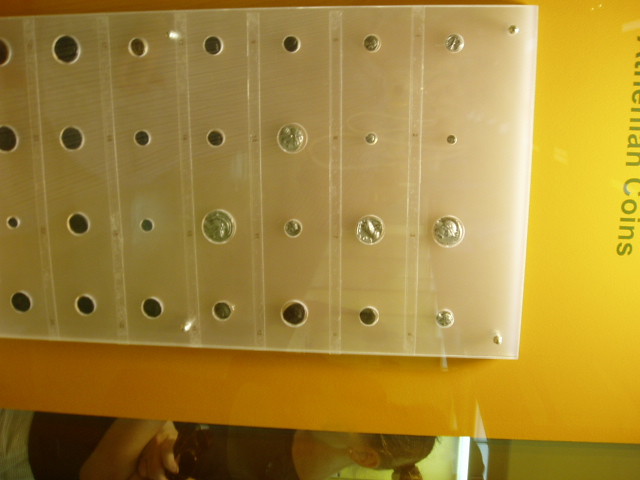This photograph displays a sideways image, likely captured in a museum, of a meticulously arranged coin exhibit set against a vibrant orange-yellow background. The coins, which include a variety of sizes and appearances—some silver, some brown or black—are housed within a clear, rectangular plexiglass case that is secured by bolts. The plexiglass case features a grid of evenly spaced holes, some of which are filled with coins. However, due to the angle and lighting, the specific details on the coins are not discernible, though a few appear to have faces on them, possibly indicating different years. The coins and holes are lined up in precise rows and columns, with these patterns becoming more spaced out as the arrangement extends. Additionally, toward the right side of the photograph, there are vertical inscriptions, read from top to bottom in the sideways image, possibly indicating the title or description of the coin collection. The photograph’s horizontal orientation also reveals a person's head at the bottom, adding a sense of scale to the exhibit.